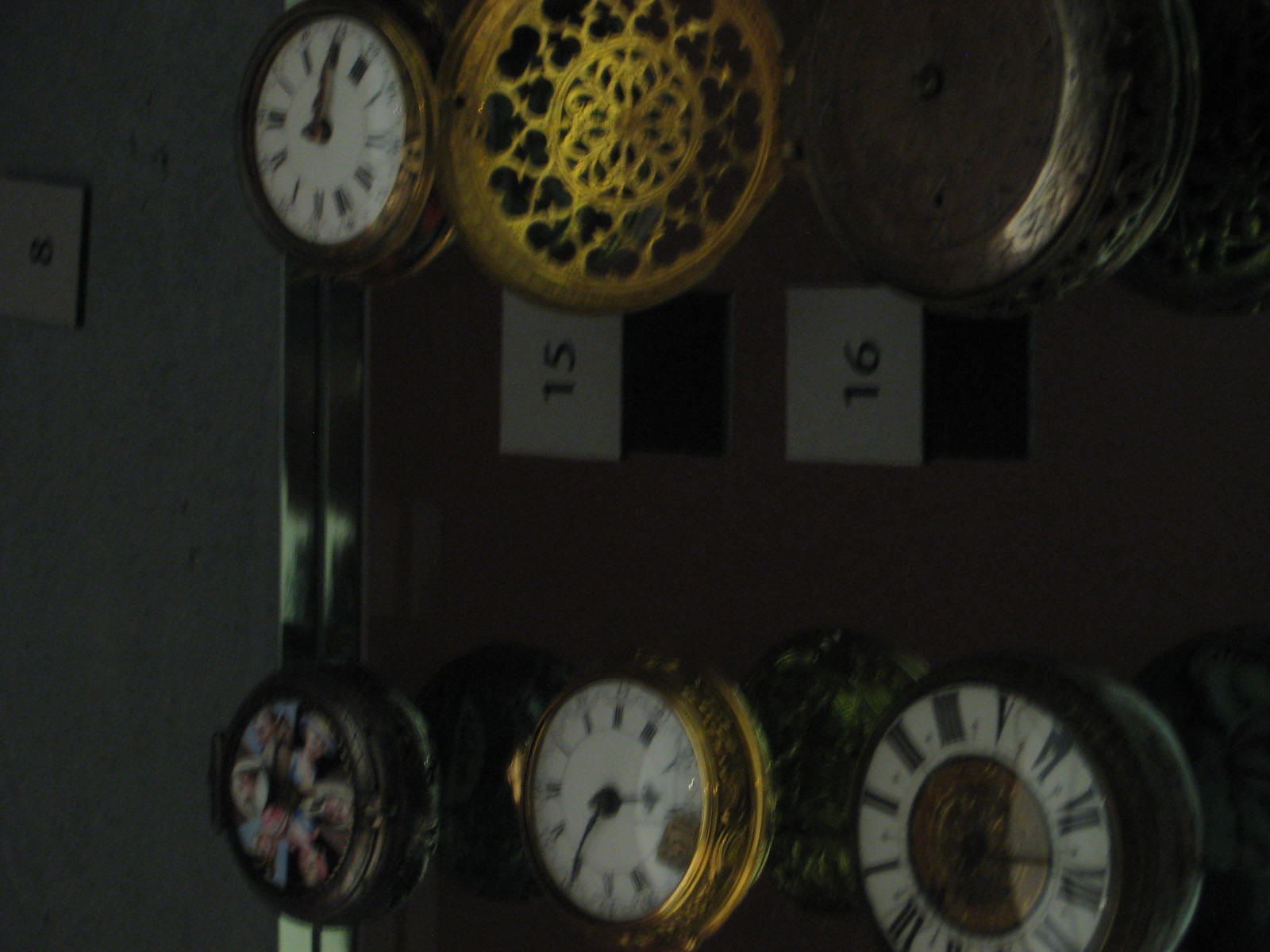This image, taken in a dimly lit room with low light illumination, showcases an arrangement of six ornate clocks mounted on a dark gray wall, potentially made of wood. The setting is minimal with focus solely on the clocks, which are aligned in two rows of three each. The upper left corner of the image features a light switch with a light-colored faceplate. 

The faces of the clocks, each displaying different times, are varied in style and material. Four clocks have white faces, mostly adorned with Roman numerals and black hands. One clock boasts a gold filigree design, and another, partially obscured by darkness, is less discernible. Among the notable details, two clocks are accompanied by the numbers 15 and 16 next to them, while another set of numbers, 8, might be present elsewhere on the wall. The clocks have a mixture of gold and silver elements, with one entirely gold clock showing the time as 12:05.

Overall, the image conveys an eclectic, almost vintage collection of timepieces that contribute to an enigmatic, almost eerie atmosphere within the room.